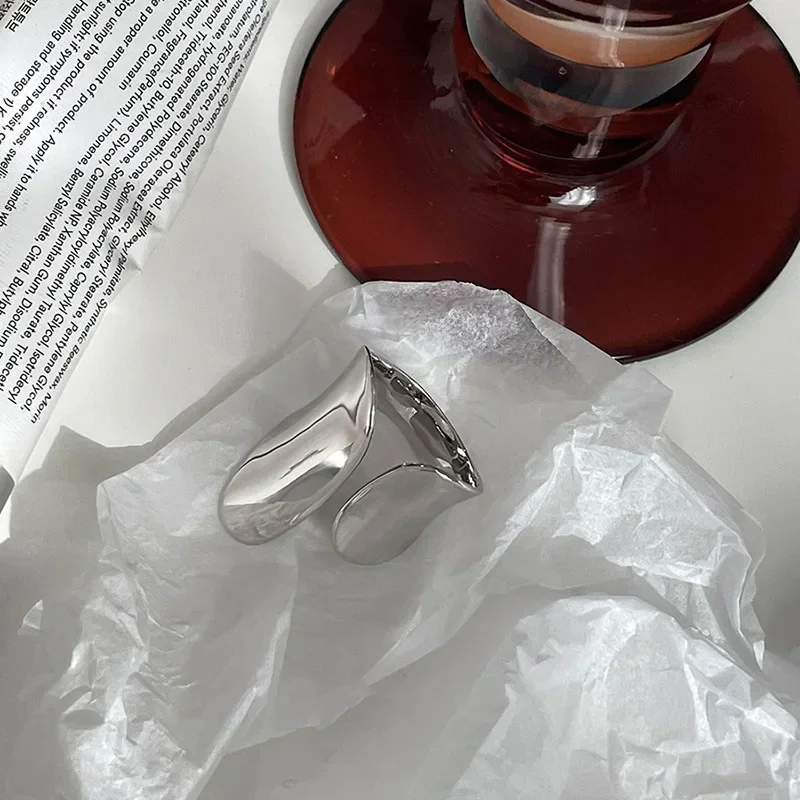The photograph depicts a meticulously arranged scene on a white table. Dominating the upper right section is a dark red, almost translucent, glass object that appears to be a large, circular coaster or base with a cylindrical column rising from its center. Resting on this glass object is a shiny black and brown coffee mug, adding a reflective element to the picture. 

In the upper left corner, there's a white piece of paper with extensive black text, possibly instructions or an article, mentioning chemicals like Butyl glycol. This paper is partially folded, contributing to a sense of casual arrangement.

The bottom half of the image showcases a piece of white, crumpled packing paper that looks soft to the touch. Placed atop this paper is a small, shiny silver object resembling a clip or a bracelet, which is longer on the left side than on the right. This silver piece curves gently, adding an element of intrigue to the photograph. 

Overall, the image presents a harmonious interplay of textures and materials, with glass, paper, metal, and ceramic elements thoughtfully positioned on a pristine white table.